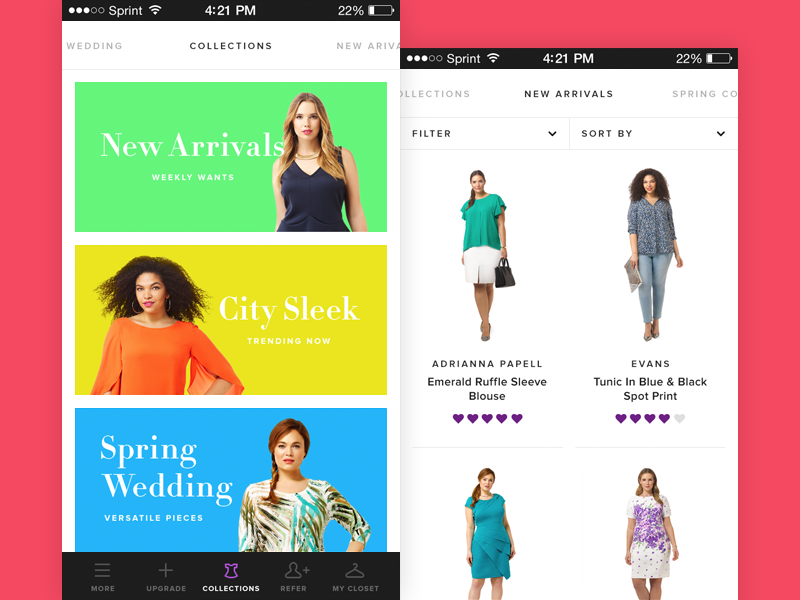This photograph features two smartphone screenshots overlaid on a pink background. The screenshot on the left is positioned slightly higher and aligned at the top, while the one on the right is staggered slightly lower, with the two touching at the center.

On both screenshots, the status bar displays "Sprint 4:21" and a 22% battery icon. The header of the left screenshot reads "Wedding Collections, New Arrivals," with "Collections" highlighted. Beneath the header, various thematic colored rectangles contain images of women:

1. A green rectangle titled "New Arrivals, Weekly Wants" features a Caucasian woman with long blonde hair, dressed in a black dress.
2. A yellow rectangle labeled "City Sleek, Trending Now" shows a light-skinned African American woman in an orange top, with frizzy hair blowing in the wind.
3. A blue panel titled "Spring Wedding, Versatile Pieces" displays a red-haired woman with braided hair.

At the bottom of this screenshot, there are options for "More Upgrade Collections, Refer in My Closet."

The right screenshot appears to be a continuation, showing a partially cut-off menu under the "Collections, New Arrivals" header. The highlighted section "New Arrivals" is centered, suggesting a menu shift when selected.

Below, there are options to "Filter and Sort By," followed by four images of women against white backgrounds:

1. A woman in an "Adriana Papel, emerald ruffle sleeve blouse" paired with a white skirt and holding a briefcase.
2. A woman in an "Evans tunic in black and blue spot print" wearing jeans and holding an item.
3. A woman in a blue dress.
4. A woman in a white and purple dress.

Underneath the top two images, the left has five purple hearts, while the right shows four or five purple hearts and a gray heart.